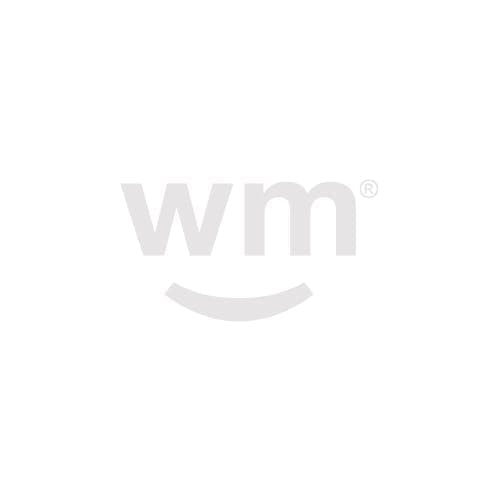The image features a logo set against a completely white background. Central to the image are the faint, almost silvery gray letters "WM," with a small, circular trademark symbol to the right of the "M." Positioned beneath the letters is a slightly curved line, reminiscent of a subtle, sideways parenthesis or the gentle curve seen in the Amazon logo's arrow, giving the impression of a mouth. This arrangement of elements— the "WM" as eyes and the curve as a smile—unintentionally creates a face-like illusion if observed for some time. The entire composition exudes a minimalist aesthetic with its very light, nearly white coloration and simple, clean design.